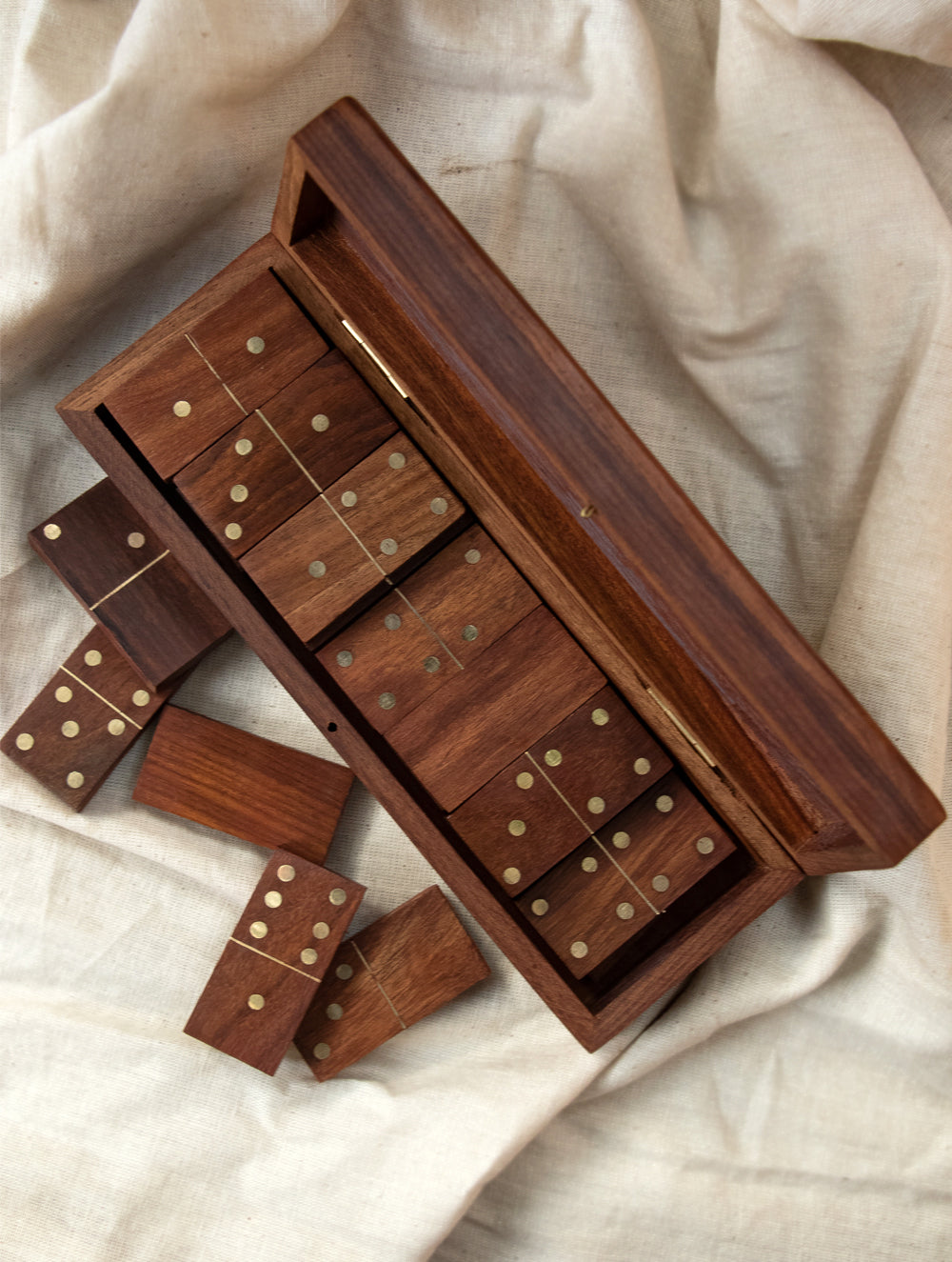The photograph showcases a custom-made wooden domino set, primarily composed of maple wood with a rich, dark brown hue and prominent natural wood grain visible throughout both the pieces and the case. The dominoes feature distinctive brass dots and lines for the numbers, creating a striking contrast against the wood. The set is partially housed in an open, slim rectangular wooden case, which matches the width of the domino pieces. Several dominoes lie outside the case, casually strewn over a ruffled linen or canvas-like fabric, adding a rustic backdrop to the polished set. The image, taken from an overhead perspective, emphasizes the high-quality craftsmanship and the elegant interplay of brown, gold, and tan colors in the scene.